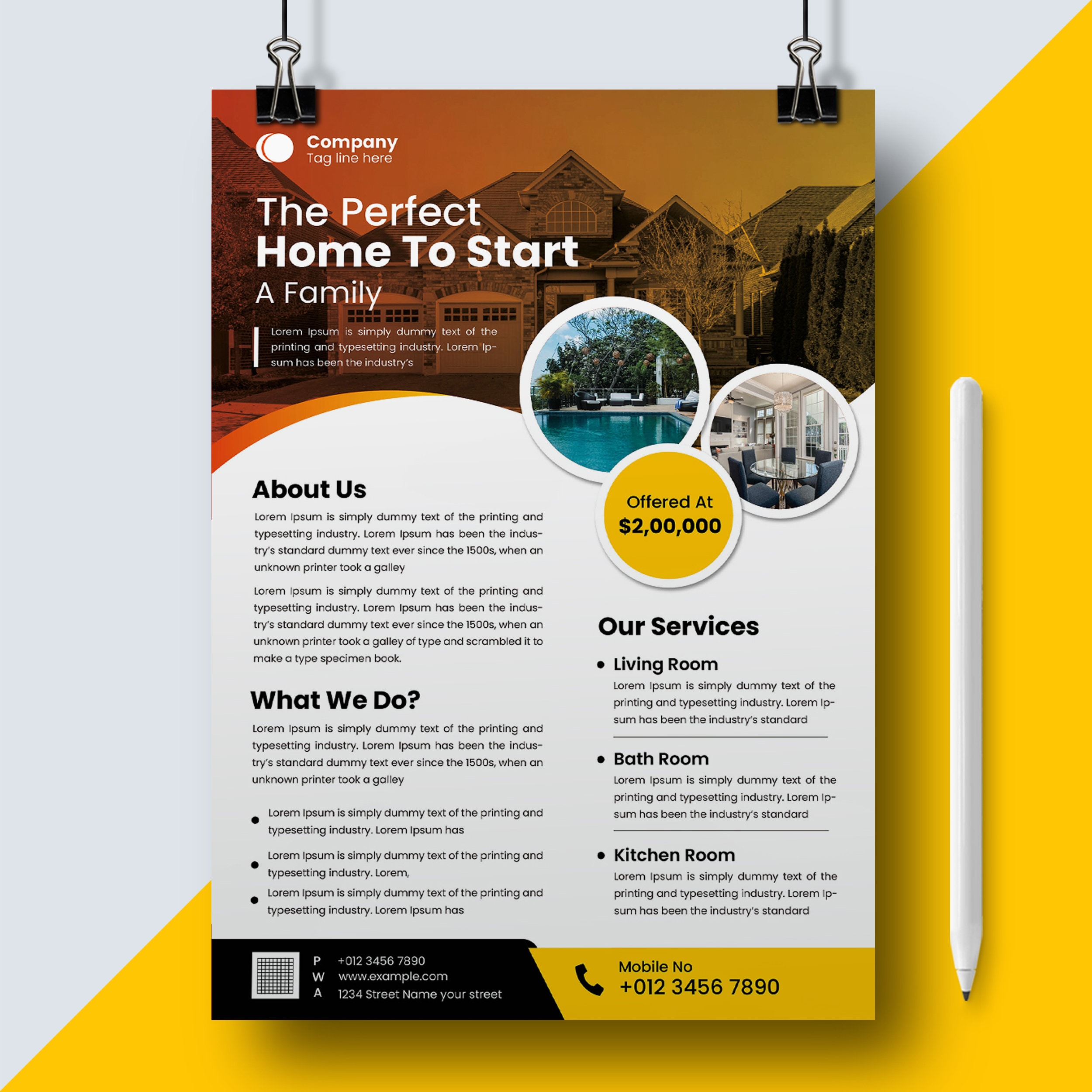The image is a large, perfectly square advertisement with a background divided diagonally from the bottom left to the top right. This creates an upper white triangle and a lower yellow triangle. The advertisement is suspended at the center, seemingly hung from the ceiling by black and silver binder clips attached to black strings. The promotional content of the pamphlet reads "The perfect home to start a family," offered at two million dollars. It features vivid colors with images including a pool and a living room. 

The text is organized into sections: "About Us" with two descriptive paragraphs, "What We Do" with a paragraph and three bullet points, and "Our Services" detailing the living room, bathroom, and kitchen with corresponding text beneath each heading. A mobile phone number, marked with a plus sign and formatted as +012-345-67890, is displayed prominently at the bottom right, against the yellow triangle background. There’s also a white pen with a black tip lying vertically on the yellow section of the background, suggesting a creative and well-thought-out design.